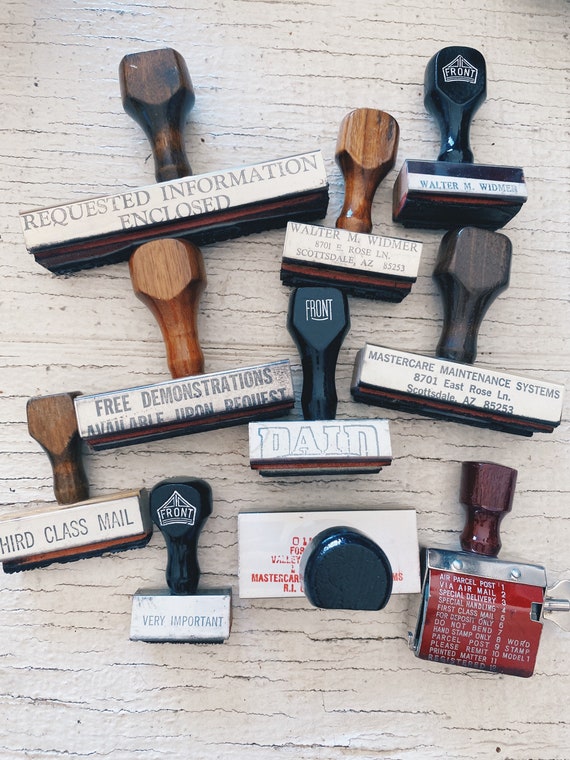This image showcases an assortment of ten vintage rubber stamps, each with a wooden handle, arranged on a light-colored wooden table. The foremost stamp in the upper left corner is the largest and bears the inscription "Requested Information Enclosed." Adjacent to it is a smaller stamp with the faintly visible text "Walter M. Windemere," and an address that hints at Scottsdale, Arizona. Below these, there is a stamp that declares "Free Demonstrations Available Upon Request," and another marked "Paid." The "Master Care Maintenance Systems" stamp includes an address, specifically 8701 East Rose Lane, Scottsdale, Arizona. Further down, a stamp labeled "Third Class Mail" and one marked "Very Important" can be seen. Another stamp standing upright is obscured, revealing only its holding knob. On the far right, there is a multi-stamp device, designed to switch between messages, including "Air Parcel Post," "Via Airmail," and "Special Delivery." Each stamp varies in size and slightly different in typography, reflecting a variety of purposes from mailing instructions to promotional notices.